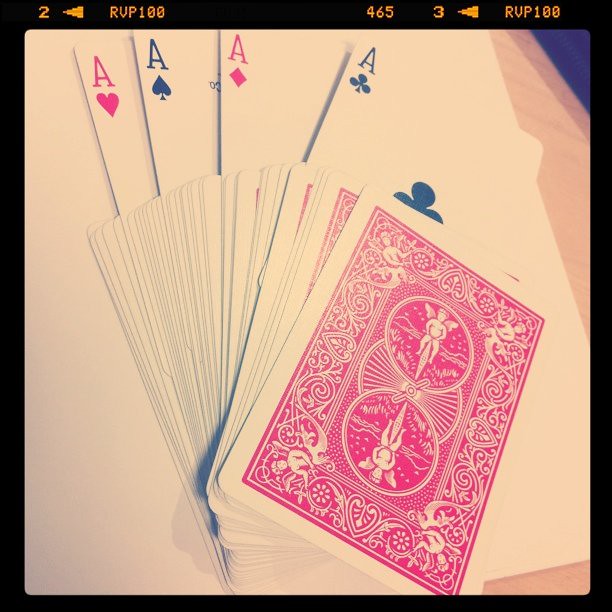The image prominently showcases a set of playing cards situated as the main focus. It is enclosed by a thin, black, square-shaped border that features yellow lettering at the top. The text includes a "2" with an arrow pointing to the right or left, followed by "RVP 100." Along the left center of the border, the numbers "465" and "3" are displayed, accompanied by another left-pointing arrow and the text "RVP 100," all in a yellowish-orange font.

The playing cards lie on a light brown wooden surface, which could be a table or floor, partially covered by a white piece of paper. On this white paper are four aces face up: the ace of hearts at the bottom, slightly overlapped by the ace of spades but leaving the heart visible. Above them, the ace of diamonds is placed with a slight overlap on the ace of spades, and the ace of clubs is spread out further on top.

A deck of playing cards with a red back design is artistically swirled around on top of these aces, creating a dynamic arrangement.